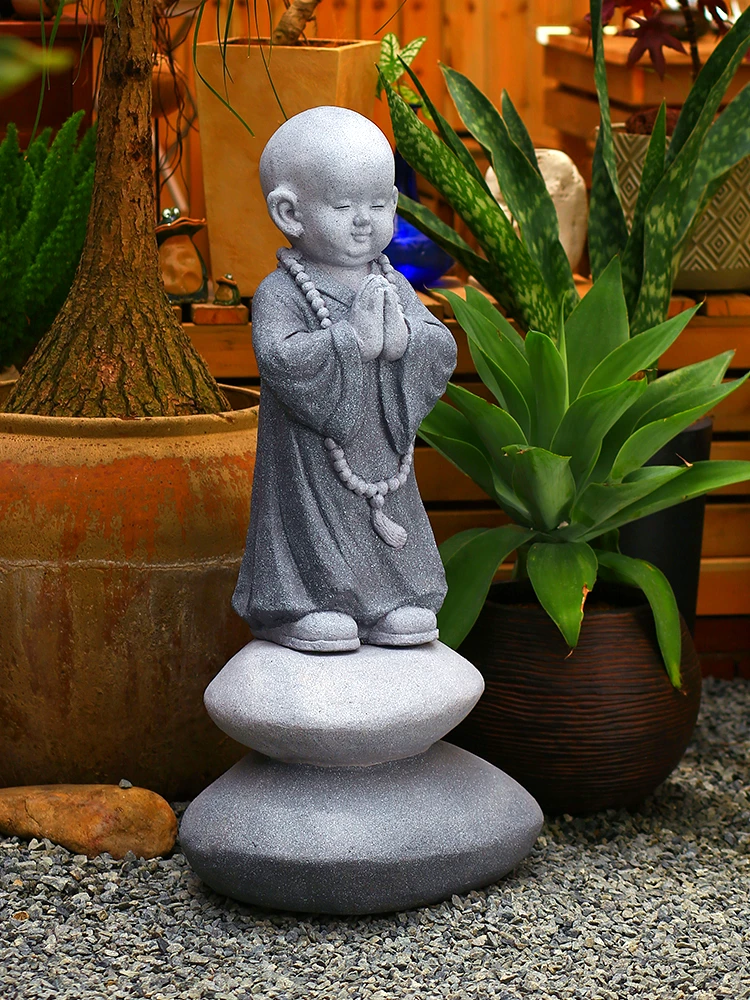The photograph, taken in portrait orientation, captures a serene garden scene centered around a small, detailed Buddhist statue. The statue, resembling a Baby Buddha, is entirely gray and stands on two smooth, stacked rocks atop a gray gravel ground. The figure is bald with a large cranium, shut eyes, round cheeks, and large ears, all contributing to its endearing, peaceful expression. The statue is dressed in a gray robe and adorned with thick, large prayer beads around its neck, with its hands folded in a prayerful gesture. To the left of the statue is a potted tree trunk, though its top is not visible, and to the right, there is a well-maintained green plant. The background features elements typical of a Zen garden, including more potted plants and hints of wooden structures such as a patio and terracotta pots, lending a tranquil, meditative atmosphere to the scene.